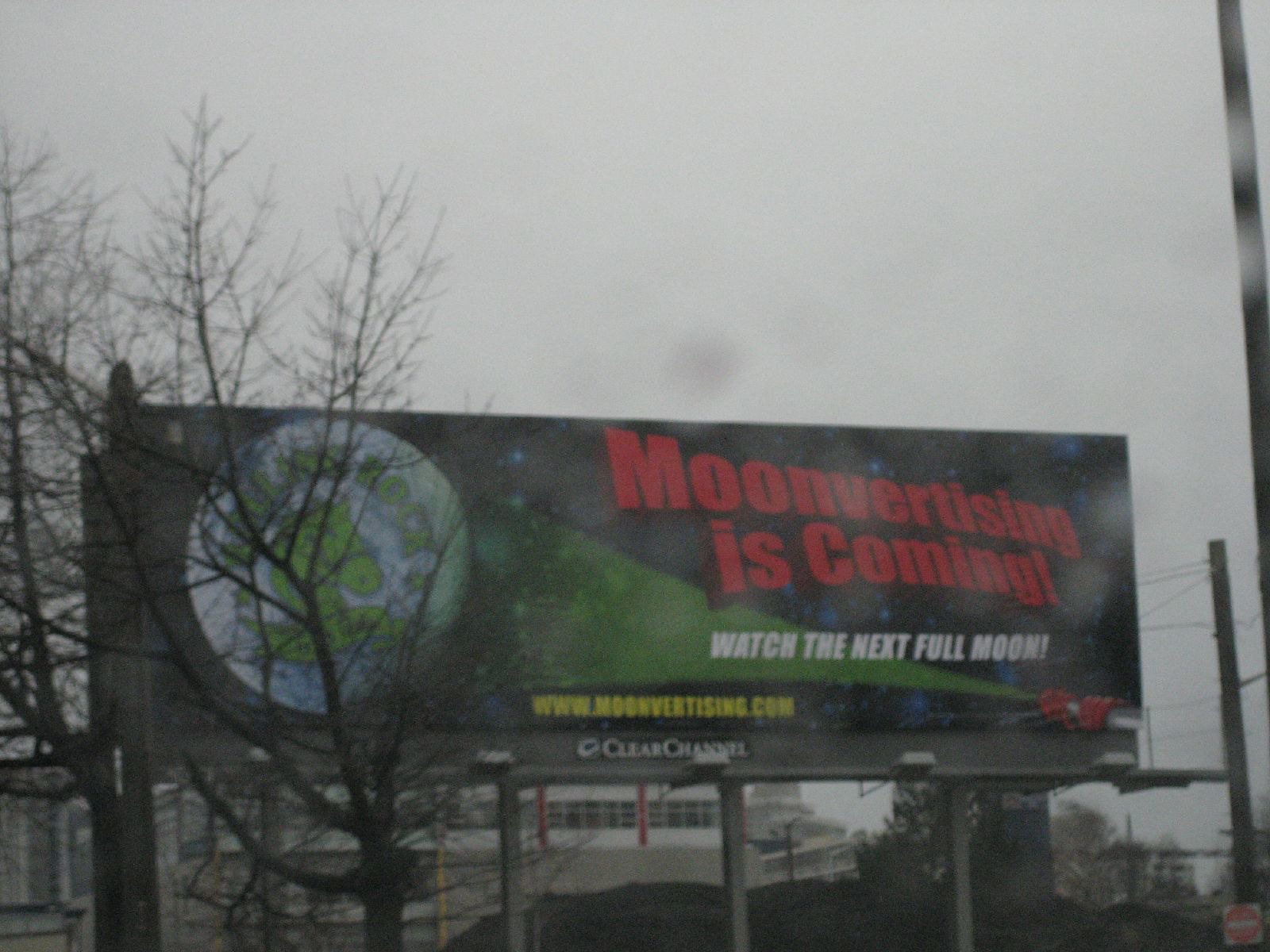The image showcases a large outdoor billboard advertisement set against a wintry, gray sky. The billboard is prominently displayed with a black background featuring bold red letters stating, "Moonvertising is coming," followed by the white text, "Watch the next full moon," and the yellow URL, "www.moonadvertising.com." Below this, in silver, is the logo for "Clear Channel." The advertisement also displays a planet with blue and green imaging, illuminated by a green light controlled by two red-gloved hands. The setting includes leafless trees on the left, gray poles supporting electrical wiring on the right, and a partially obscured white and gray building in the background, which could be a stadium. The scene is acknowledged as very wintery and dreary, further emphasized by the bare branches and the overall gray tone. The billboard itself is supported by six pillars and positioned in close proximity to a telephone pole.